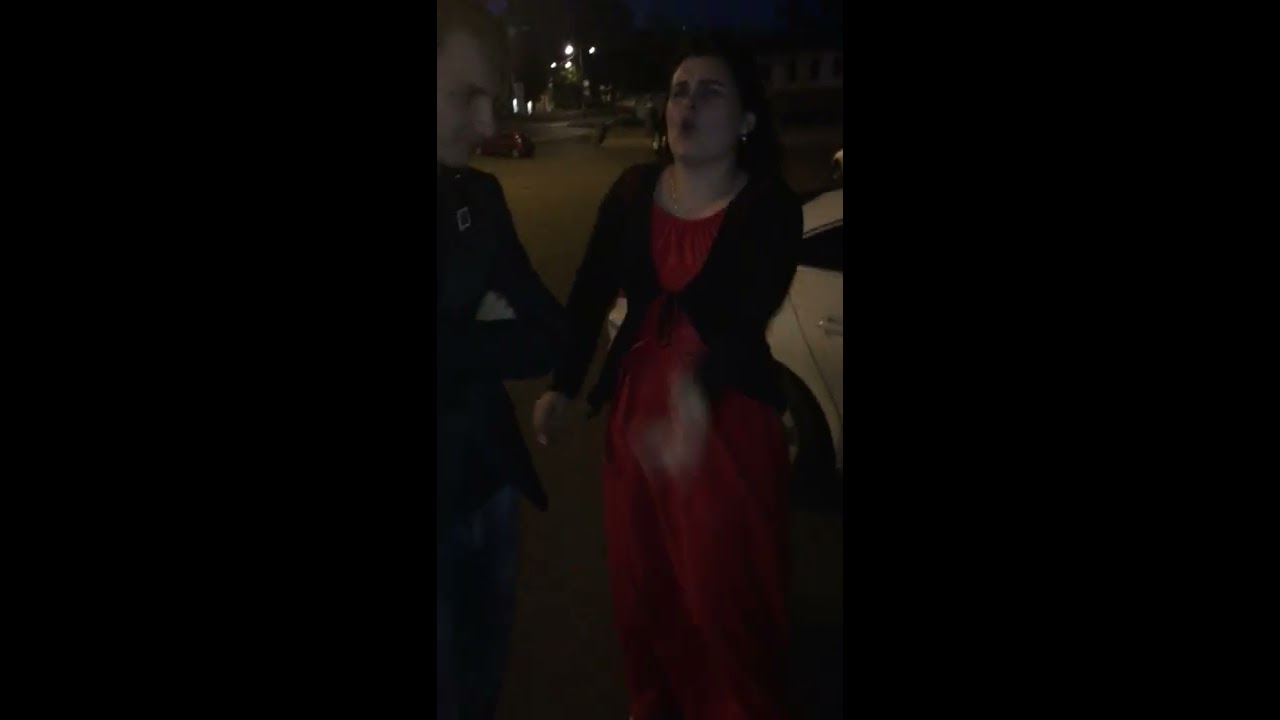A nighttime city street forms the backdrop for this central photograph of a triptych, flanked by two plain black panels. The image captures a young Caucasian woman with dark hair, wearing earrings, a long red dress, and a black coat or cardigan. She stands slightly tilting her head back, her lips pursed in an expression that seems pained, her eyes closed. Her right hand is raised, caught in a blurred motion. To her left, partially visible and slightly off-frame, is a man with blondish or brown hair, arms crossed, clad in a dark jacket and blue jeans. He appears contemplative, looking sideways and downward. The street is dimly lit, with streetlights and cars providing sparse illumination. A white car is parked behind the woman, its door handle and part of its body visible, while further back, hints of a red car and perhaps some passing pedestrians add to the bustling, albeit shadowy, urban night scene.